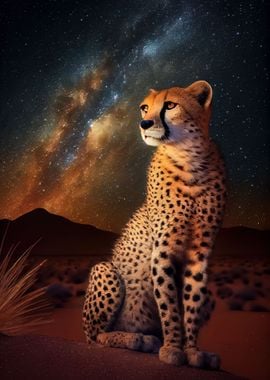In this digitally generated illustration, a majestic leopard with orange fur, black spots, and a white underbelly is depicted resting on its hind legs with its front legs fully extended, causing its upper body to rise prominently. The leopard, possibly mistaken for a cheetah, has a distinctive black nose and is positioned on a rock, gazing off towards the left. The setting appears to be a desert, marked by sandy terrain and scattered small plants. In the background, a shadowy mountain looms under a dramatic night sky. This sky is a mesmerizing blend of dark blue, grey, golden brown, and yellow hues, illuminated by countless stars. Portions of the sky also exhibit glowing streaks, suggesting a hint of celestial light or possibly the emergence of dawn.